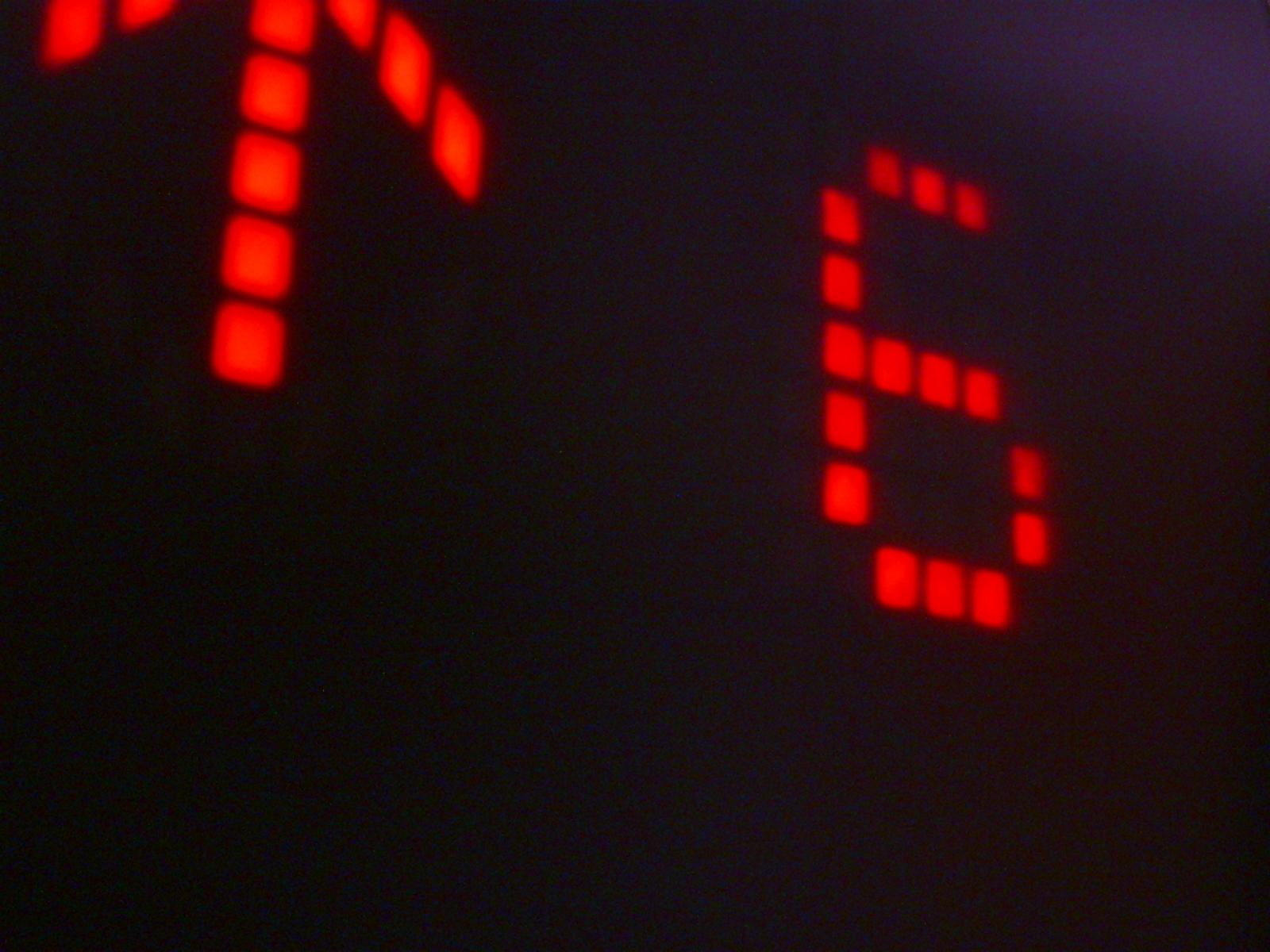The image depicts a very close-up view of a digital display set against a completely black background, reminiscent of a sign one might find at an airport terminal or train station departure board. In the top left corner, an arrow composed of red LED squares points upwards, while to its right, a large number "6" is similarly formed by red LED squares. The digit "6" is intricately constructed from a precise arrangement of 16 red lights. While the image's background is uniformly black, the top right section subtly transitions to a dark purple hue, possibly due to lighting or screen irregularities. Overall, the image's simplicity highlights only these red LED components against the stark black backdrop.